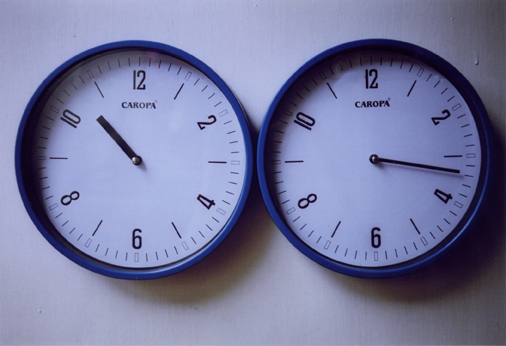The image features two blue circular clocks positioned side by side against a white background. Both clocks have a blue rim with indented white faces that display black numerals and markings, showing only the even numbers: 12, 2, 4, 6, 8, and 10. The left clock indicates a time of approximately 10:52, with a thick, wide hour hand and no visible minute hand. The right clock displays 3:18, featuring only a minute hand. Both clocks prominently display the word "CAROPA" in bold, black capital letters beneath the number 12.